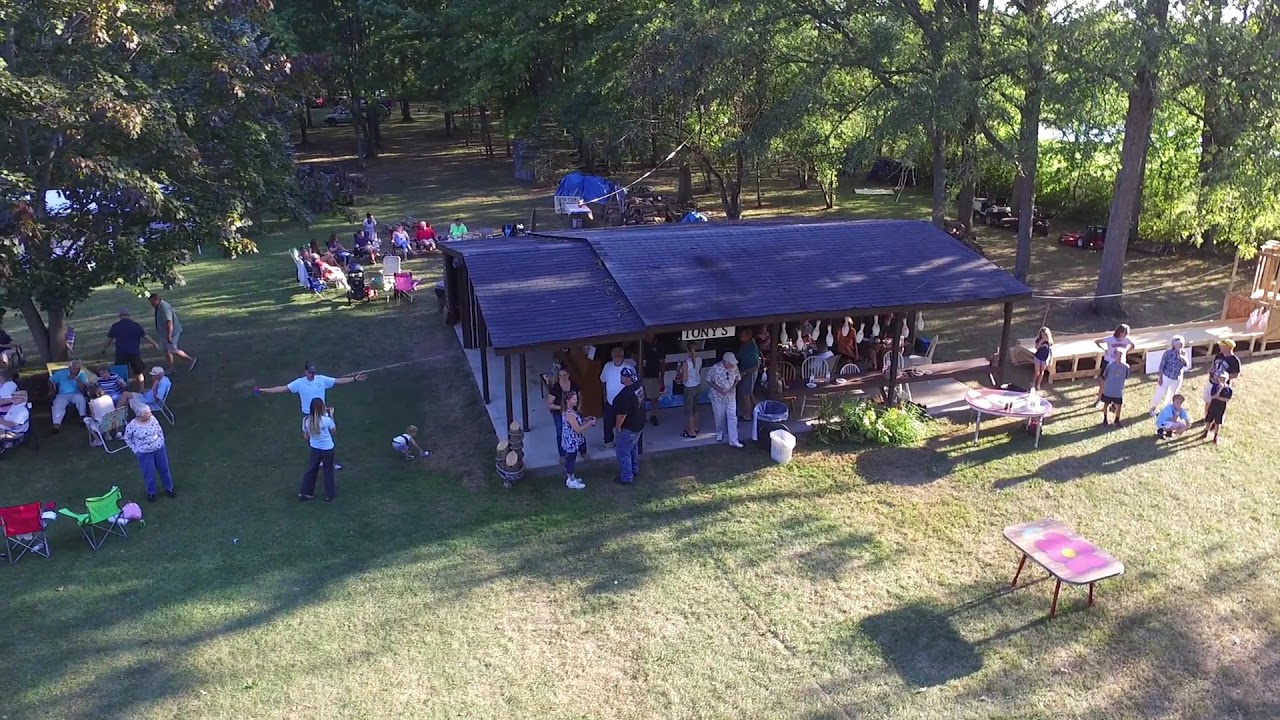The photograph presents an overhead view of "Tony's," an outdoor pavilion with a bluish-gray roof, located in a lush, green recreational area. The pavilion, centrally positioned in the image, has several people standing underneath its roof and numerous others gathering around it. A sign that reads "Tony's" hangs prominently from the roof. Around the pavilion, there is a vibrant green grassy lawn bordered by a grove of tall trees, offering shade where more individuals are gathered. To the right of the image, people are seen standing and chatting in the sunshine near a paved area with a bench. In the lower right corner, there's a table with a pink flower design. The left lower corner features a red and a green lawn chair. Overall, the bright daylight highlights the various activities and interactions happening in this lively outdoor setting, giving the impression of a communal celebration or event.